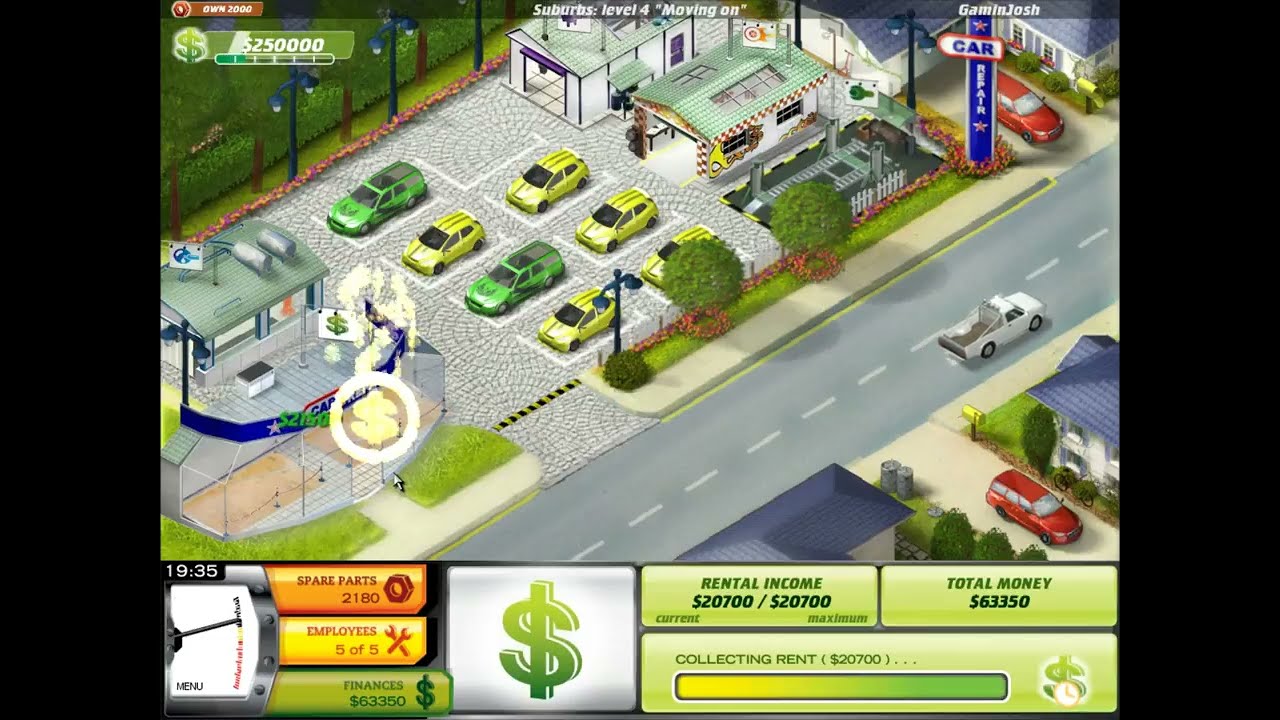The image is a screenshot from a video game featuring a bird's-eye view of a small town street corner. In the center, noticeable from the sky, is a car rental lot filled with green and yellow-green cars, a red car, and a white truck driving on a light gray road with dashed white lines. Off to the side of the road, there's an establishment with "Car Repair" written in white on a blue sign, flanked by red stars at the top and bottom.

Both the left and right sides of the screenshot are bordered by thick black lines framing the central content. In the upper right-hand corner, the name "Gaminjosh" appears in white print. At the far left, a green dollar sign displays a monetary value which seems to be $250,000, partially underlined by a green bar.

At the bottom part of the screen, the game interface features several blocks of information. On the left, "Spare Parts" marked with a bolt icon lists a value, "Employees" with wrenches crossing each other shows another figure, and "Finances" highlighted by a large dollar sign indicates $63,350. To the right of it, "Rental Income" is displayed as 20,700/20,700 within a green bar, with "Collecting Rent" shown above it. Above these details, there are numbers in white text on a black background, specifically, "1935".

Background visuals include a nearby parking lot, additional buildings that seem to be garages, grassy patches with trees, shrubs, and growing flowers. Across the street, white houses with blue rooftops add to the suburban setting. The video game's interface includes colored indicators and icons, emphasizing various shades including green, yellow, red, and blue, giving a comprehensive view of the simulated environment.